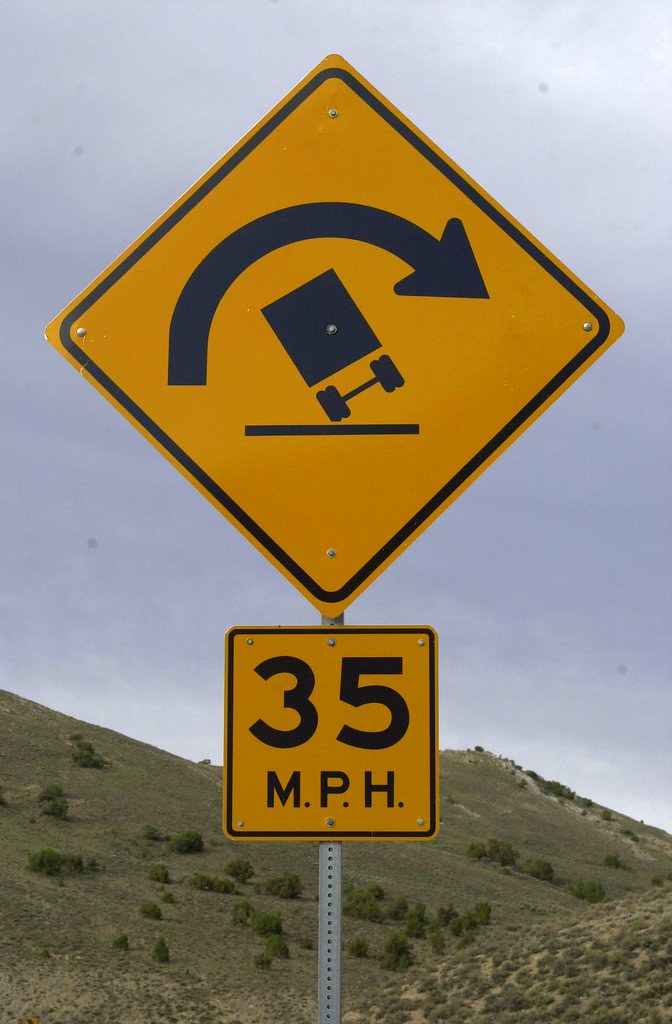A detailed image of a road sign prominently displayed against a backdrop of hilly terrain characterized by green bushes and a mix of brown and gray soil. The foreground features a reflective metal pole supporting a pair of signs: a yellow diamond-shaped sign with a black border, illustrating a tractor trailer tipping to the left and an arrow pointing to the right, indicating a potential hazard for large trucks taking sharp turns at high speeds. Below it, a square yellow sign marked "35 MPH" in black font clearly indicates the speed limit. The sky above is a blend of blue and slight cloudiness, adding to the scenic yet cautionary nature of the setting.